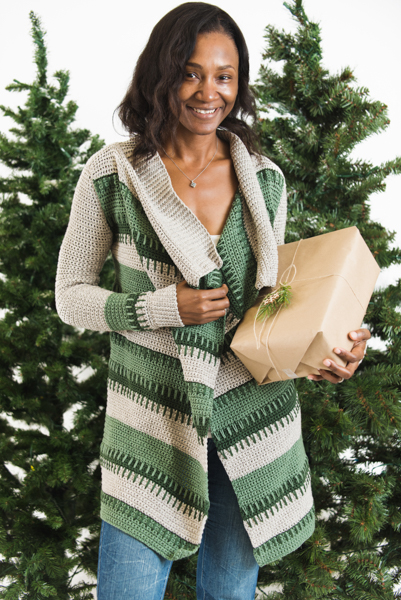This photograph captures a beautifully smiling, young Black woman in her late 20s, exuding festive charm. She stands before two green, undecorated, fur-like Christmas trees, with a plain white background enhancing the holiday atmosphere. Her dark brown, shoulder-length hair frames her face softly. She is dressed in a stylish, long, beige and green striped sweater with a wide, open collar and long sleeves, complementing her blue jeans. Beneath the sweater, she wears a simple white tank top, paired elegantly with a delicate necklace. In her arm, she holds a neatly wrapped brown parcel, adorned with green, leafy ribbon details. The woman's radiant smile and relaxed pose, clutching her sweater, add to the warm and inviting holiday spirit of the scene. Merry Christmas!